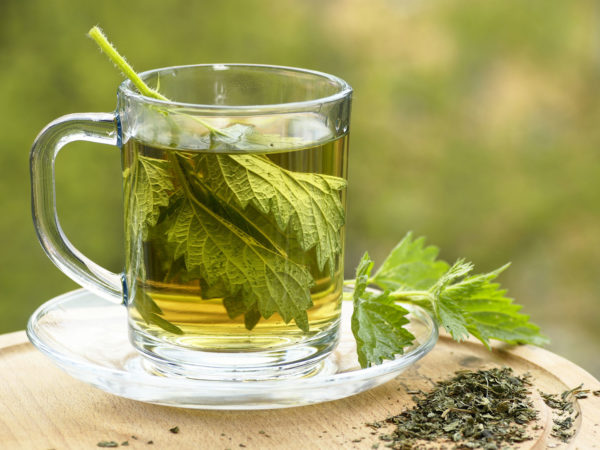This color photograph showcases a rustic outdoor setting with a small circular wooden table or stand as its focal point. Positioned centrally on the stand is a clear glass saucer and an accompanying mug, which is also made of glass. The mug contains a yellowish liquid, likely tea, into which a branch with green, sawtooth-edged leaves is immersed. Beside the mug, on the saucer, is another sprig of similar green leaves. To the right on the wooden table, there's a noticeable pile of dried leaves, adding to the natural theme of the image. The table itself is marked by a distinct groove around its edge. The background features out-of-focus greenery with hints of trees and grass, enhancing the serene, nature-filled ambiance of the scene.